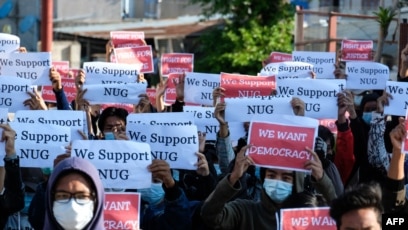The image captures a vibrant and crowded protest scene featuring a diverse group of masked men and women holding up various signs. Dominantly, there are white signs with dark lettering that read "We support NUG" and red signs with white borders that declare "We want democracy." The protestors' faces are largely obscured either by the signs they're holding or by their face masks. A notable feature in the background is a green tree, hinting at a public space in possibly an Asian country. Additional visual elements include an old building, a fence, and possibly a small shack or shed. Some individuals are also seen wearing hats or hoodies. The entire setting is under daylight, adding to the clarity and vibrancy of the scene. The lower part of the picture features white letters spelling out "AFNP."